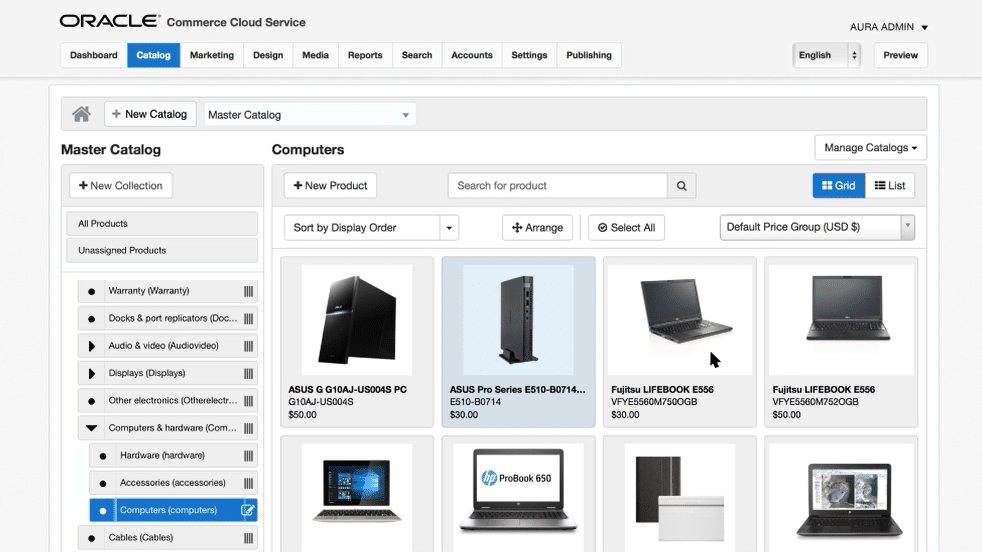The image is a capture of a website for Oracle Commerce Cloud Service, showcasing various pieces of hardware available for purchase. The hardware displayed includes a tower, a mini tower, four laptops, a server, and an additional laptop, all presumably available for purchase. The website features a master catalog to facilitate browsing, though the image is too small to discern the specifics of the tabs clearly. However, general categories such as displays, hardware, audio, and docking are mentioned. The section currently displayed falls under 'computers.' At the top of the webpage, several nearly readable tabs are visible, including options like Marketing, Device, Media, Report, Search, Account Settings, and Publishing. This indicates that the platform likely serves as a comprehensive hub where users can purchase a variety of equipment directly from Oracle.